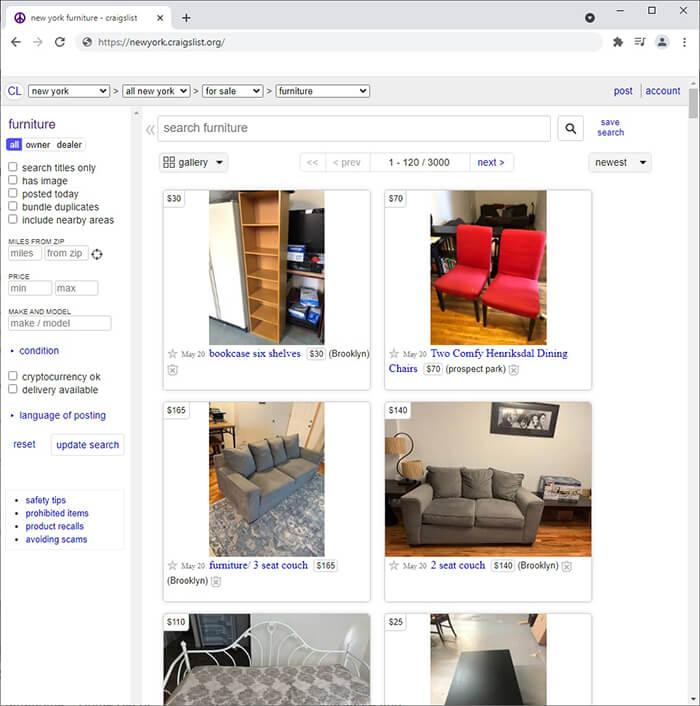This is a detailed screenshot taken from the Google Chrome web browser displaying the Craigslist website, specifically the New York section of Craigslist under the 'for sale' category, focused on furniture listings. The user has selected "New York" and "all New York" for the search parameters but has not applied specific filters such as price or condition. The results show six furniture items with accompanying images: a bookcase, two chairs, a sofa, another sofa, a bed, and a table. The listed prices range from $25 to $165. However, the bottom two items (the bed and the table) are partially cut off, obstructing the view of their exact names and specific locations within New York. The other items clearly display their locations, including areas such as Brooklyn and Prospect Park.